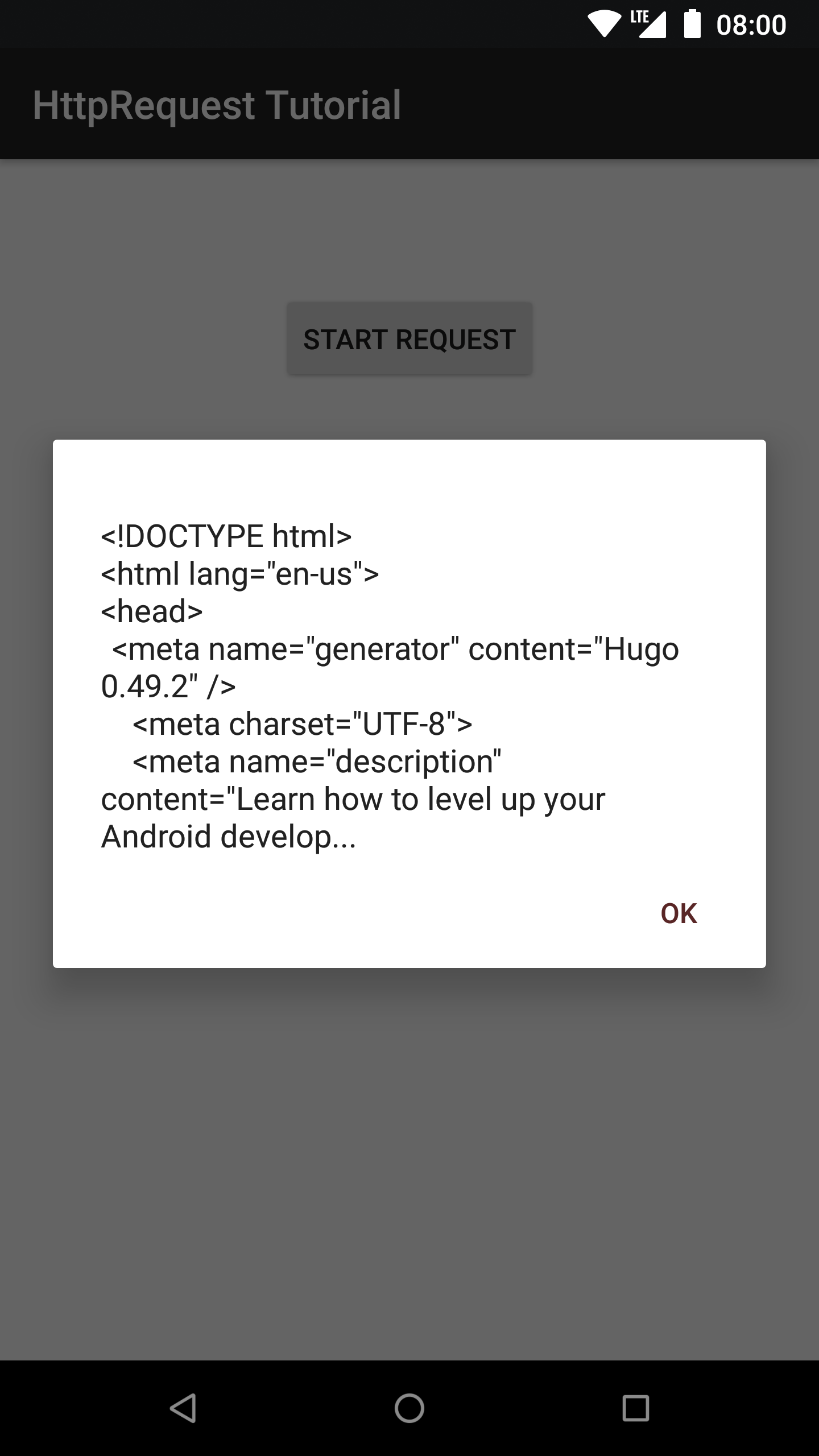The screenshot captures a mobile phone interface displaying a web browser error message at 8:00 AM. The screen features a top black bar with indicators for full Wi-Fi, LTE cellular service, and a fully charged battery. Below, on a grayed-out white background, a central gray pop-up box with black text reads "Start Request."

Inside the pop-up, a text block appears, starting with unusual characters and HTML elements, suggesting a coding or rendering error. Among the visible text are tags such as `<!DOCTYPE html>`, `<html lang="ENG">`, `<head>`, `<meta name="generator" content="Hugo 0.92.49.2">`, `<meta charset>`, `<meta name="description" content="How to order, level up, Android developer">`. The word "God" is notably displayed at the top of this block, followed by nonsensical characters including a sideways arrow and exclamation mark.

Towards the bottom right corner of the pop-up box, there’s an "Okay" button, likely to dismiss the error message. The base of the screen includes a black bar with three gray navigation icons: a triangle pointing left (likely the "Back" button), a circle (possibly the "Home" button), and a square (probably the "Recent Apps" button). The entire scene appears to be a captured moment of a technical issue encountered during web navigation on an Android device.